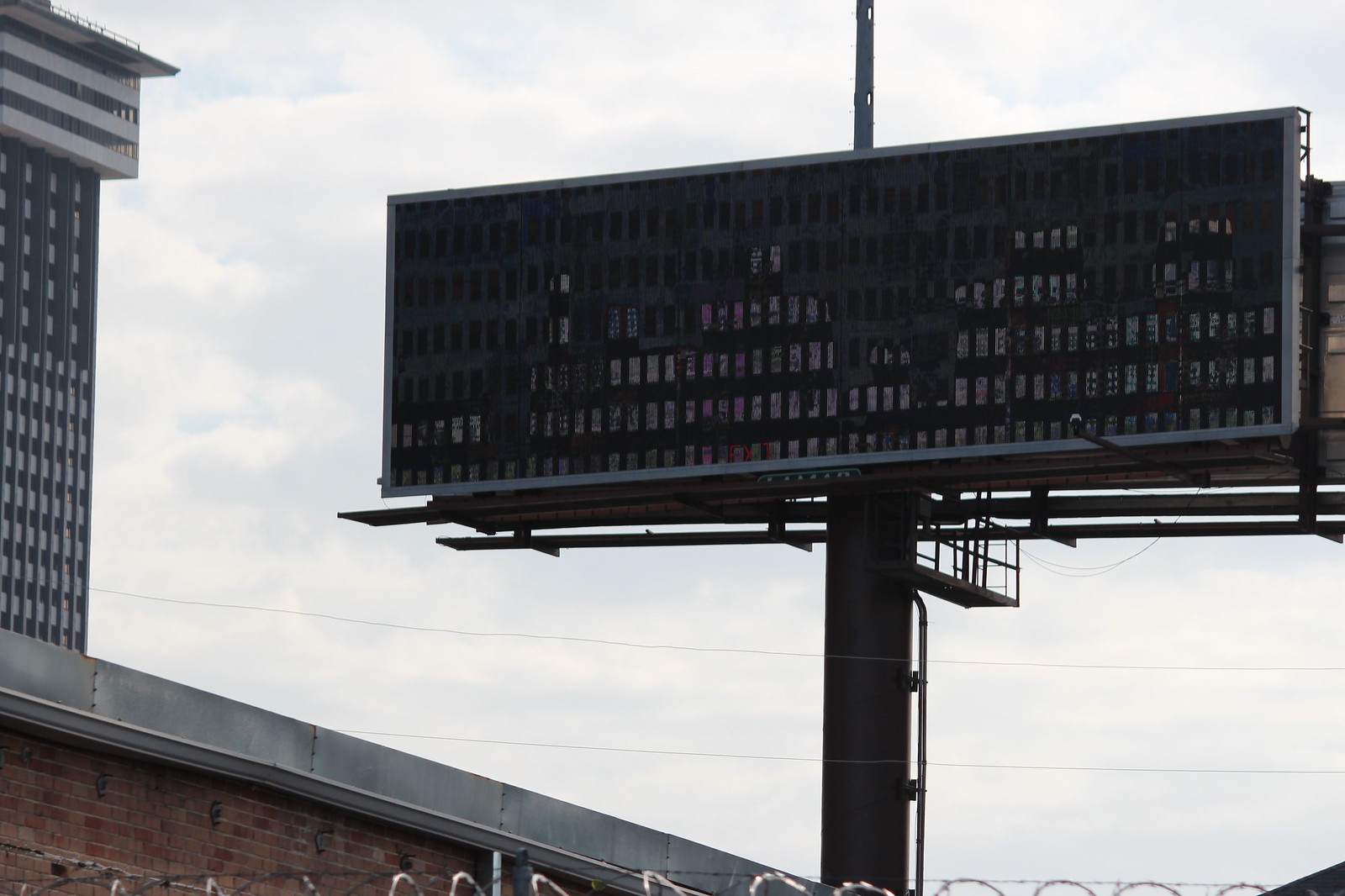This outdoor color photograph captures a cityscape under a cloud-covered, light blue sky. Dominating the left side of the image is a tall building with several stories, featuring numerous windows and an upper section extending outward, possibly an observation deck. In the midground, a smaller brick building with a metal roof stretches to the center of the photograph. A wire fence, topped with spiraled barbed wire and a gray metal barrier, runs along the bottom edge. Central to the image is a large black electronic signboard mounted on a tall pole. The signboard, which appears to have tiny holes with some colored fillings, does not display any text or images. The scene is devoid of people, animals, plants, and vehicles, set against an overcast sky with blue hues shining through the clouds.